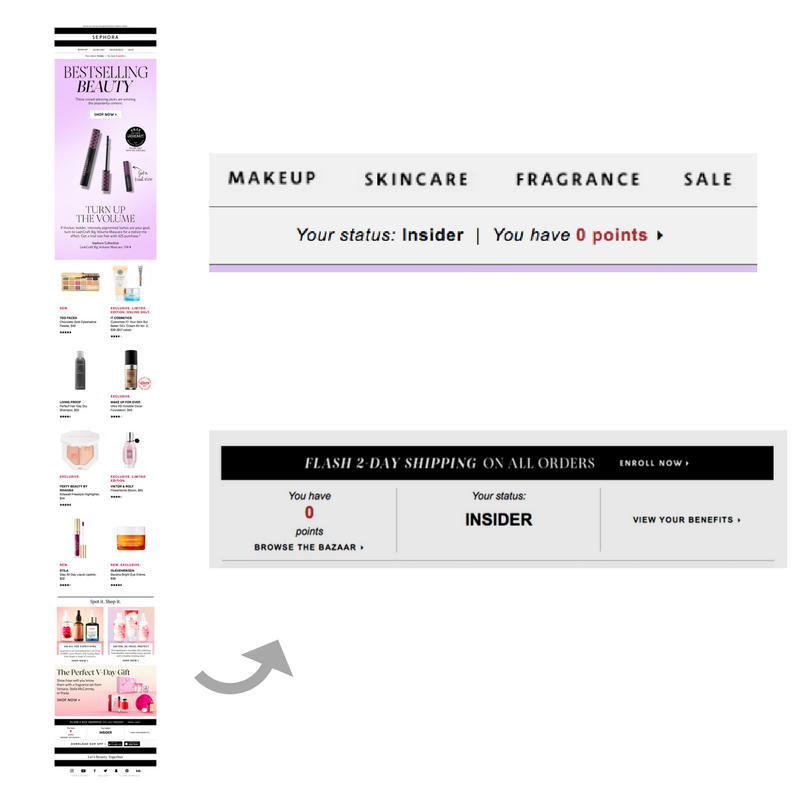This visually complex image is divided into several distinct sections, each conveying different information related to beauty products and services:

On the right side of the image:
- A vertical, rectangular section features the word "SEPHORA" in bold black letters on a white background, framed by two thick, horizontal black lines.
- Adjacent to this is a vertical light purple section displaying the phrase "BEST-SELLING BEAUTY" in all caps black letters, surrounded by various makeup items.
- Below this, the phrase "TURN UP THE VOLUME" is inscribed in black, with smaller, less readable text underneath.
- Continuing down are two columns of small makeup product images, each with brief black text descriptions. Near the bottom of the first column, a gray arrow directs attention to the second column.

At the top of the second column:
- A light gray horizontal rectangle features the words "MAKEUP," "SKINCARE," "FRAGRANCE," and "SALE" in all caps black letters.
- Below this, the image outlines user status details: "YOUR STATUS" in black font followed by "INSIDER" in bold black all caps; "YOU HAVE" in black, followed by "ZERO" in red, and "POINTS" in black.
- Another horizontal light gray rectangle further down displays "FLASH TWO-DAY SHIPPING ON ALL ORDERS" in all caps gray writing on a black background, with "ENROLL NOW" in smaller fonts below it.

On the left side, there's additional user status information:
- "YOU HAVE" in black, "ZERO" in red numbers, and "POINTS" beneath it.
Additionally, "BROWSE THE BAZAAR" is bolded.
- In the middle, it reiterates "YOUR STATUS:" in bold black letters, followed by "INSIDER" in all caps black letters, and "VIEW YOUR BENEFITS" in smaller all caps black fonts.

The detailed presentation and well-structured layout effectively highlight various promotional content and user-specific information.